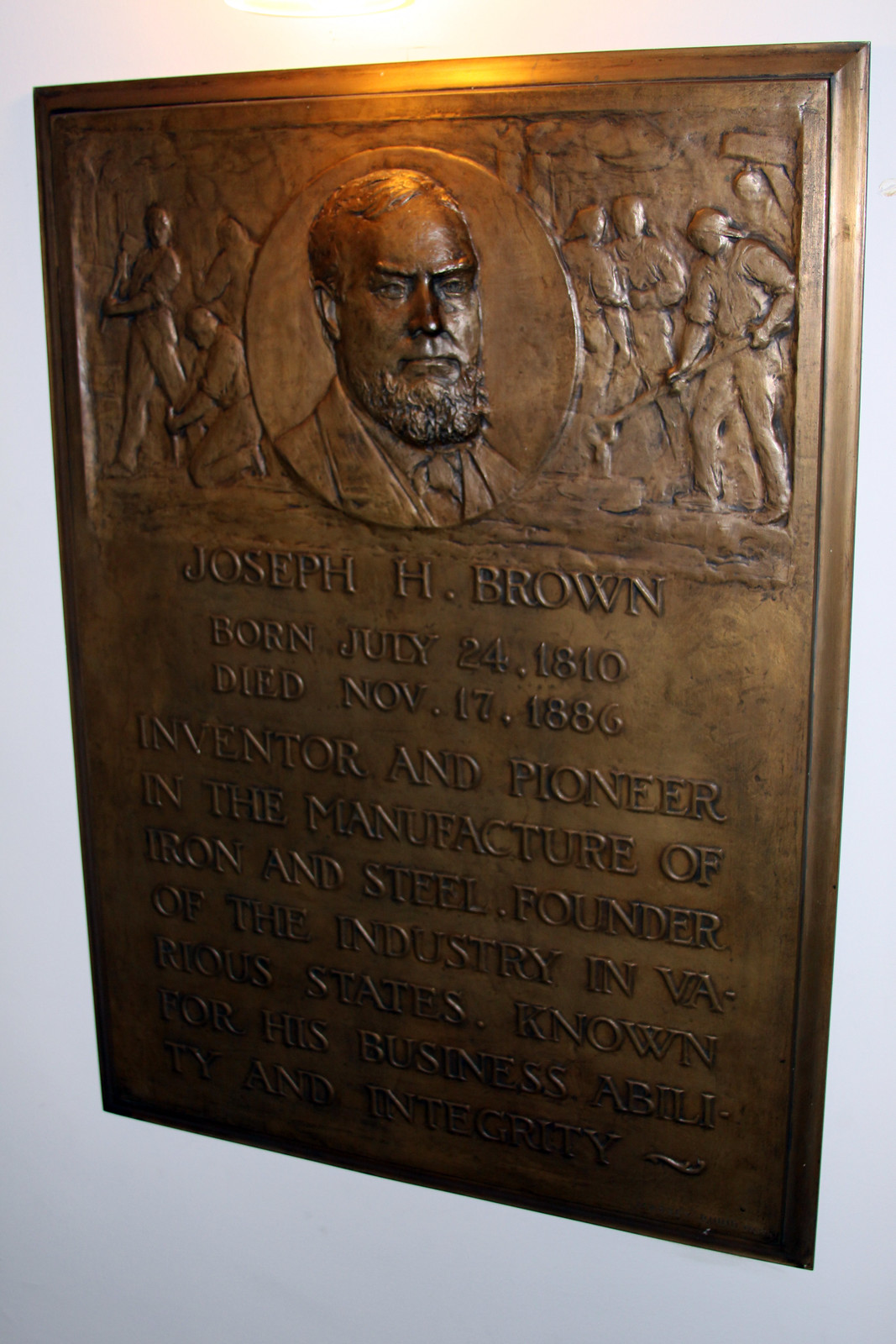The image features a bronze plaque mounted on a solid white wall, illuminated by a light source from above. At the top center of the plaque is a circular inset with a detailed portrait of a man identified as Joseph H. Brown; he is depicted with short hair, a beard without a mustache, and is wearing a suit jacket with a tie. Flanking the central portrait on both the left and right are intricate carvings of miners at work, possibly in a mine shaft, symbolizing the industrial context associated with the man. The inscription beneath the portrait reads: "Joseph H. Brown, born July 24, 1810, died November 17, 1886, inventor and pioneer in the manufacture of iron and steel, founder of the industry in various states, known for his business abilities and integrity." The plaque's lower part is somewhat obscured in darkness, adding to the solemnity of the tribute. The setting suggests an indoor location, possibly a museum, where this piece serves as a commemorative artifact. The predominant colors in the image are white, bronze, and hints of yellow and orange from the lighting.